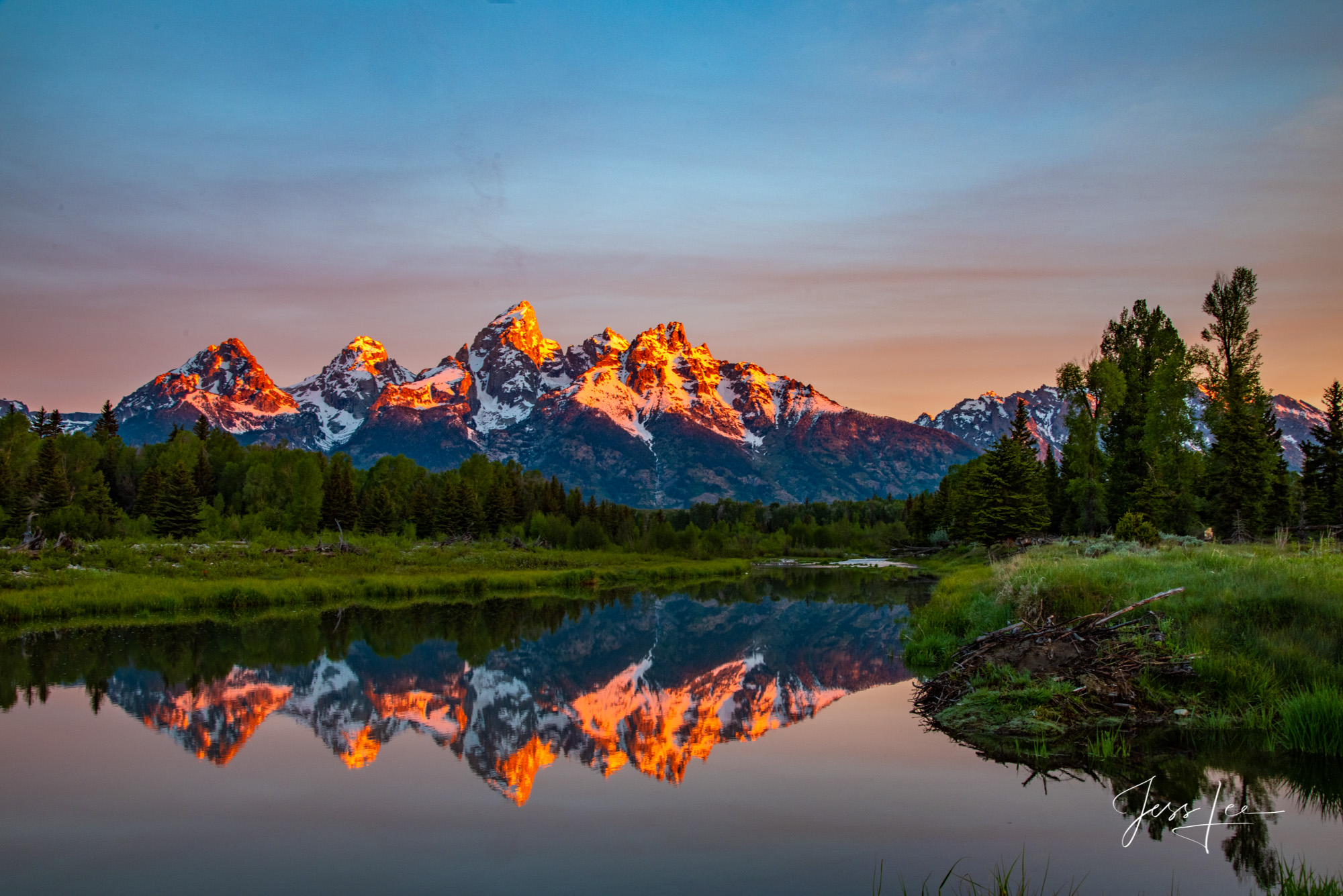The image is a stunning photograph of an untouched, serene natural landscape that could easily grace the pages of National Geographic. At the forefront is a tranquil pond acting like a mirror, perfectly reflecting the majestic mountains in the background. These snow-capped peaks stretch almost the entire width of the image, their tips glowing a brilliant orange and yellow from the setting or rising sun, lending them an almost ethereal, fiery appearance. Surrounding the pond is a lush expanse of greenery, with an abundant forest of tall, vibrant trees adding depth and life to the scene. The sky above is mostly clear with a hint of scattered clouds, bathed in the soft, warm light of the golden hour. The stillness of the water and the rich colors of the landscape create a peaceful, almost pristine atmosphere, suggesting an undisturbed wilderness that invites exploration and reflection. Notably, there are no people in sight, and the only human touch is the artist’s signature, "Jess," subtly placed at the bottom of the photograph.